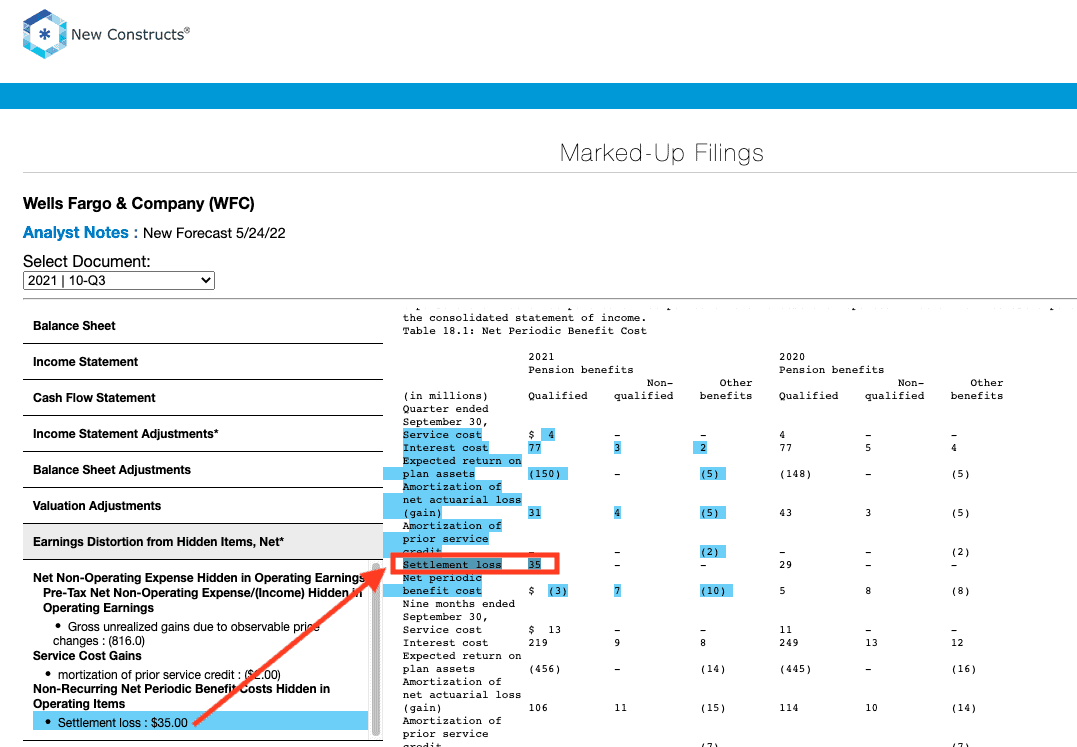The image depicts a chart, possibly related to financial data for Wells Fargo & Company. The background is entirely white, and there is no indication of a web address or other elements to confirm that it's a webpage. At the top left corner, the text "New Constructs" is visible. Below it, there is a light blue banner line followed by the text "Marked-Up Filings."

The chart includes various highlighted elements, predominantly in bright blue. In the first column on the left, a "Settlement Loss of $35" is prominently highlighted in bright blue. A red arrow connects this to a second column where the same "Settlement Loss of $35" is boxed off in red. The chart is part of an analyst note, offering a forecast dated May 24, 2022. Multiple items across the chart are highlighted, indicating significant points, all marked in the same bright blue color.